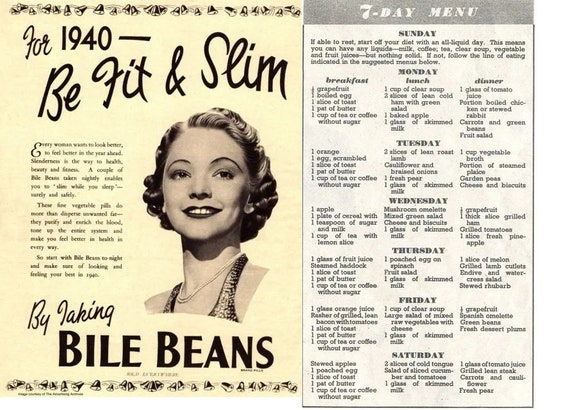This horizontal, rectangular image appears to be from an old magazine, as suggested by the vintage style of the woman's short, curly hair. The image is divided into two sections. The left side features a light beige background with bold, capitalized text stating, "For 1940 – be fit and slim by taking BILE BEANS." Beneath this headline, there's an image of a smiling woman and a justified paragraph extolling the benefits of these vegetable pills, claiming they not only help disperse unwanted fat but also purify and enrich the blood. The paragraph begins with "Every woman wants to look better, to feel better in the years ahead."

On the right side, set against a gray and white background, there is a detailed seven-day menu plan aimed at complementing the bile beans regimen. Each day of the week is centered and listed in sequence: Sunday through Saturday, with respective meal plans for breakfast, lunch, and dinner under each day. For example, Monday's menu includes breakfast options like grapefruit, a boiled egg, toast with butter, and a cup of tea or coffee; lunch features clear soup, lean cold ham with green salad, a baked apple, and skim milk; dinner consists of tomato juice, boiled chicken or stewed rabbit, carrots, green beans, and fruit salad. The detailed meal plans continue similarly for the rest of the week.